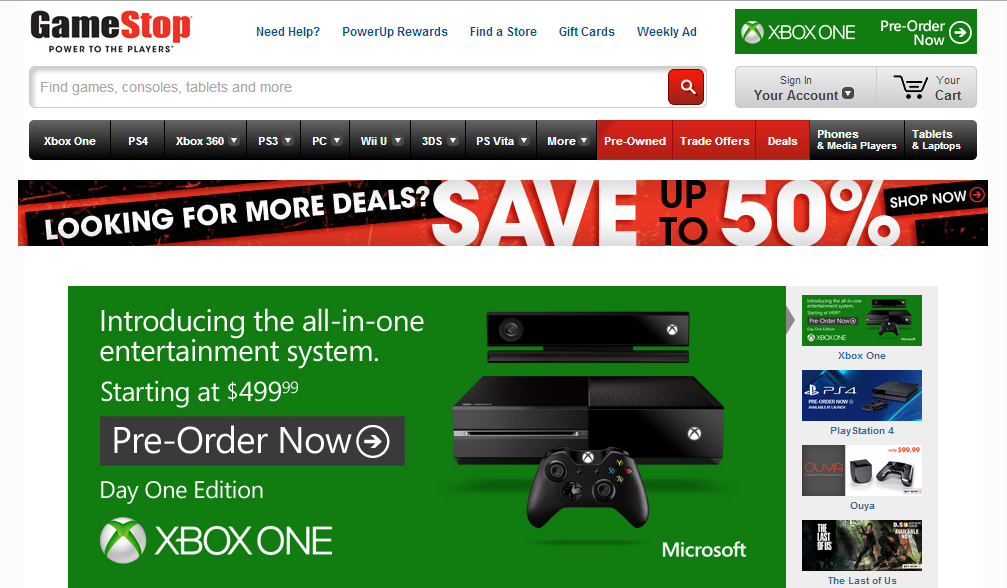In the upper left-hand corner of the image, the GameStop logo is prominently featured, displaying the slogan "Power to the Players," with "Stop" in red and the rest of the text in black. Immediately to the right of the logo, blue text reads: "Need Help? Pop Rewards, Find a Store, Gift Cards, Weekly Ad."

Below this text, there's a green search box where users can enter queries such as "find games, consoles, tablets, and more." A red button with a magnifying glass icon is at the end of the search bar. To the right of this search box, there are two additional boxes: one for signing into your account, indicated by a downward-pointing arrow, and the other for accessing your cart, represented by a shopping cart icon.

Below these features, the navigation bar consists of black boxes, each labeled with different categories: "Xbox One," "PS4," "Xbox 360," "PS3," "PC," "Wii U," "3DS," "PS Vita," and "More." Each category is separated by a small airplane icon pointing downwards. Additionally, there are three red boxes labeled "Pre-Owned," "Trade Offers," and "Deals." Further down, categories for "Phones & Media Players," "Tablets & Laptops" are visible.

Centered on the page, a prominent red banner with white text announces: "Looking for more deals? Save up to 50%! Shop Now."

Directly below this banner, a large green box introduces the all-in-one entertainment system, stating: "Introducing the All-In-One Entertainment System starting at $499. Pre-order now – Day One Edition Xbox One," accompanied by an image of an Xbox One console and controller.

To the side are additional banner ads for products like the PlayStation 4, OUYA, and The Last of Us, each associated with corresponding images for visual appeal.